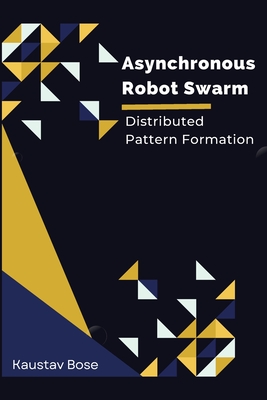The image is a meticulously designed cover of a college textbook titled "Asynchronous Robot Swarm," written in white with a yellow underline beneath it. Below the underline, it states "Distributed Pattern Formation." The author's name, "Kaustav Bose," is in white text positioned in the bottom left-hand corner. The book cover features a complex pattern of geometric shapes—primarily triangles in shades of yellow, blue, and white—creating an intricate fractal design. A prominent, larger blue triangle resides at the bottom left, with an even bigger yellow triangle positioned above it. The background is a dark blue, adding depth and contrast to the vibrant shapes and white text, resulting in a visually compelling and modern aesthetic.